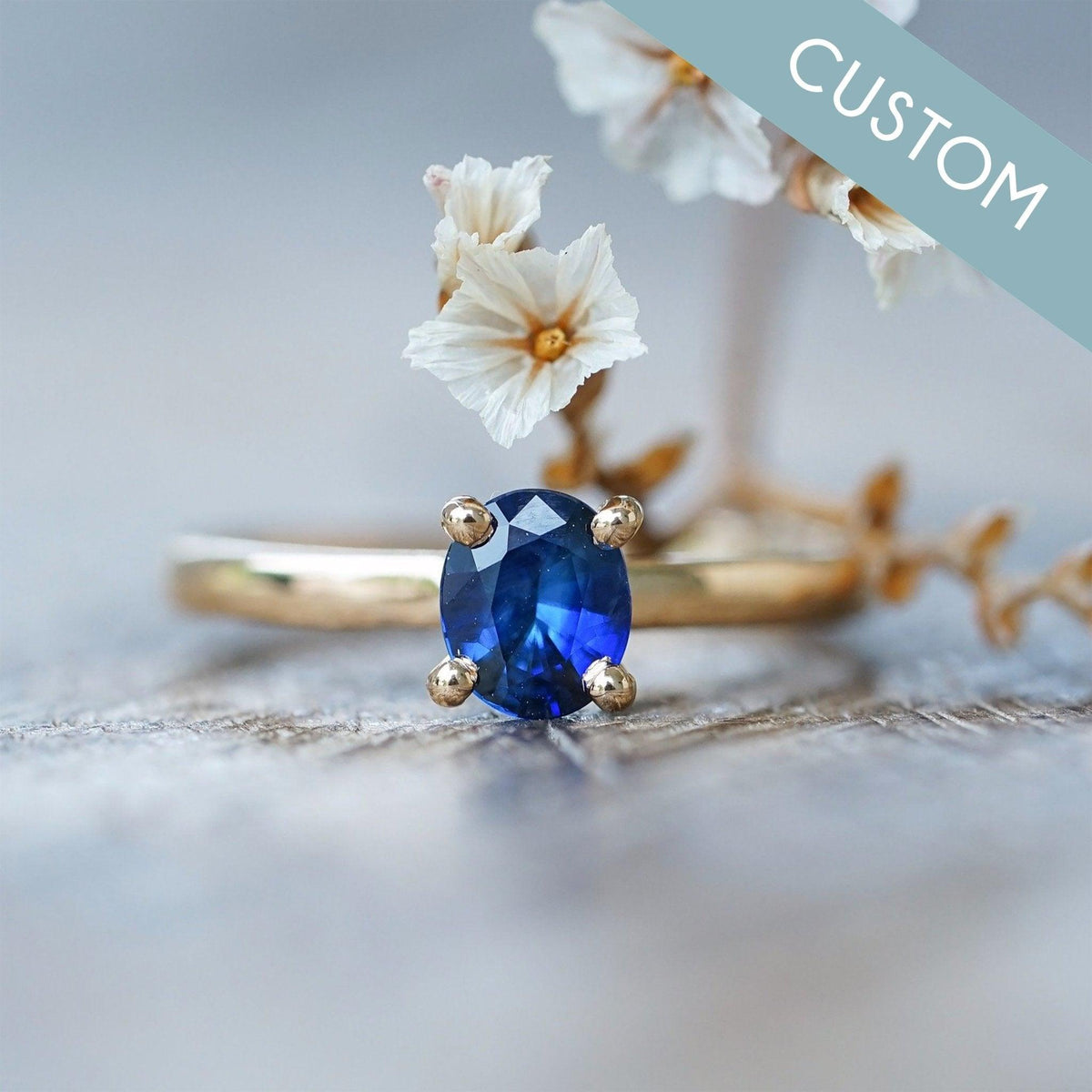This professionally posed and digitally edited full-color photograph features a striking close-up of a dark blue, oval-shaped gemstone set in an elegant gold ring. The four golden prongs securing the medium-blue stone are prominently displayed, while the slender gold band fades into the blurred background. The image is vertically rectangular with no border, shot indoors under artificial light. Decoratively arranged white flowers with brown and yellow centers are situated behind the ring, adding a delicate touch to the composition. In the upper right-hand corner, a greenish-blue diagonal banner reads "CUSTOM" in bold white capital letters, enhancing the image's polished and catalog-like presentation.